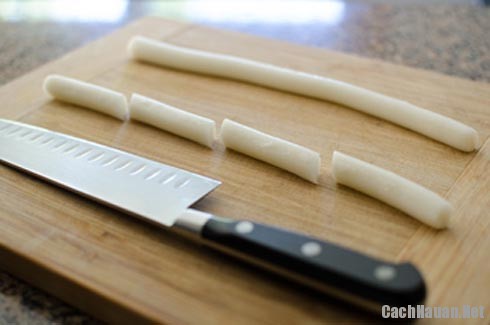The image displays a close-up of a pale, thick wooden rectangular chopping board with a natural wood grain. On the chopping board lies a prominently sharp-looking metal knife. The knife features a dark handle with three silver rivets, and its silver blade is slightly notched. Positioned diagonally, the knife's handle is on the right side of the board. To the right of the knife are two long, cylindrical, off-white strips, which could be string cheese or dough for breadsticks. The strip in the foreground is cut into four equal lengths, while the one in the background remains intact. This setup is placed on a tan and black speckled marble countertop, with a soft light reflecting from a window in the background.